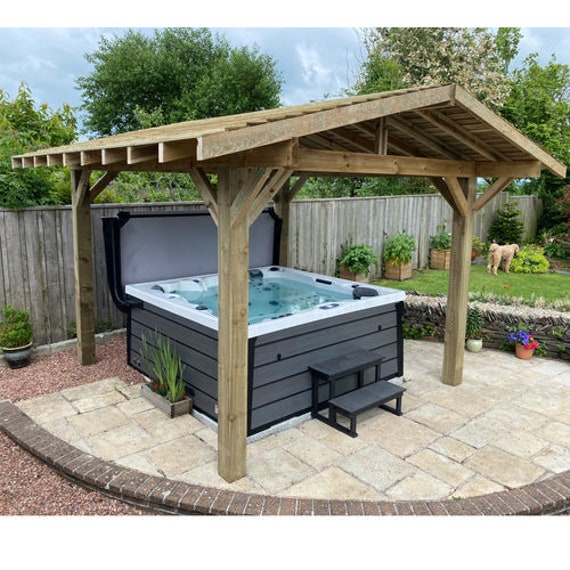In this image, we observe an outdoor setting featuring a dark grey wooden-patterned jacuzzi installed in a well-maintained backyard. The jacuzzi, designed to accommodate up to four people, is surrounded by a wooden structure supported by four slats, creating a protective roof-like covering to shield against rain or sun. This structure resembles a small pavilion or bodega. The jacuzzi sits prominently in the center of the scene, partially covered by its extended lid, with a water-filled interior.

The backyard is enclosed by a wooden picket fence, demarcating the property from adjacent areas. The landscape is dotted with neatly arranged tiles and various potted plants, contributing to a well-kept appearance. The grass is bright and lush, enhancing the garden's overall aesthetic. Several bushes and trees occupy the background, adding a touch of greenery and seclusion to the space.

Notably, a brownish dog is seen nipping at a shrub near the fence, seemingly exploring the garden area. Above, the sky is overcast with clouds, casting a soft light over the scene, further accentuating the serene and cozy atmosphere of this private outdoor retreat.